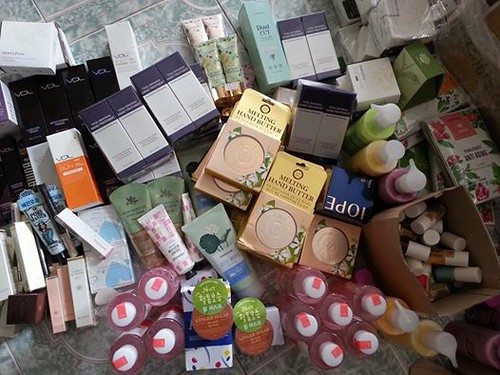The image depicts a large collection of beauty products, seemingly of Japanese or Korean origin, although there may be some American products included as well. The assortment features at least 30 different types of products, each represented by multiple units, suggesting they could be items for sale or part of a bulk purchase.

The products are meticulously yet somewhat haphazardly arranged on a light blue tiled floor, with tiles measuring about 12 by 12 inches and displaying a faint pattern. The items are grouped in an organized manner but give an impression of controlled chaos.

Several brand names and product labels are visible. A yellow box labeled "Melting Hand Butter," likely containing hand lotion, stands out among the collection. Nearby, a blue box bearing the upside-down letters "I-O-P-E" can be seen. Towards the top of the arrangement, there are four black boxes labeled "V-D-L" or possibly "V-C-L." Below these, an additional product from the same brand appears in orange and white packaging. Flanking this orange and white box are six navy blue and white boxes, arranged in groups of four and two.

The array features a vast variety of products with labels in foreign languages, making it difficult to identify all the items. Despite the language barrier and the small size of some texts, the collection is impressive and visually intriguing, hinting at a treasure trove of beauty essentials.